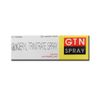The image showcases a box packaging for Glycerol Trinitrate Spray, positioned centrally against a stark white background. The packaging is divided into two sections: the left side features a light gray background with black sans serif text stating "GLYCEROL TRINITRATE SPRAY," "0.4 MILLIGRAMS PER DOSE," "200 METER DOSES," and "NO CFC, NO PROPELLANT" highlighted in red. The right section is a yellow rectangle containing two smaller rectangles; the upper one is red with white sans serif text reading "GTN," and the lower one is black with white text stating "SPRAY." This detailed and symmetrical design, devoid of other objects, makes the packaging's informational content the focal point of the image.